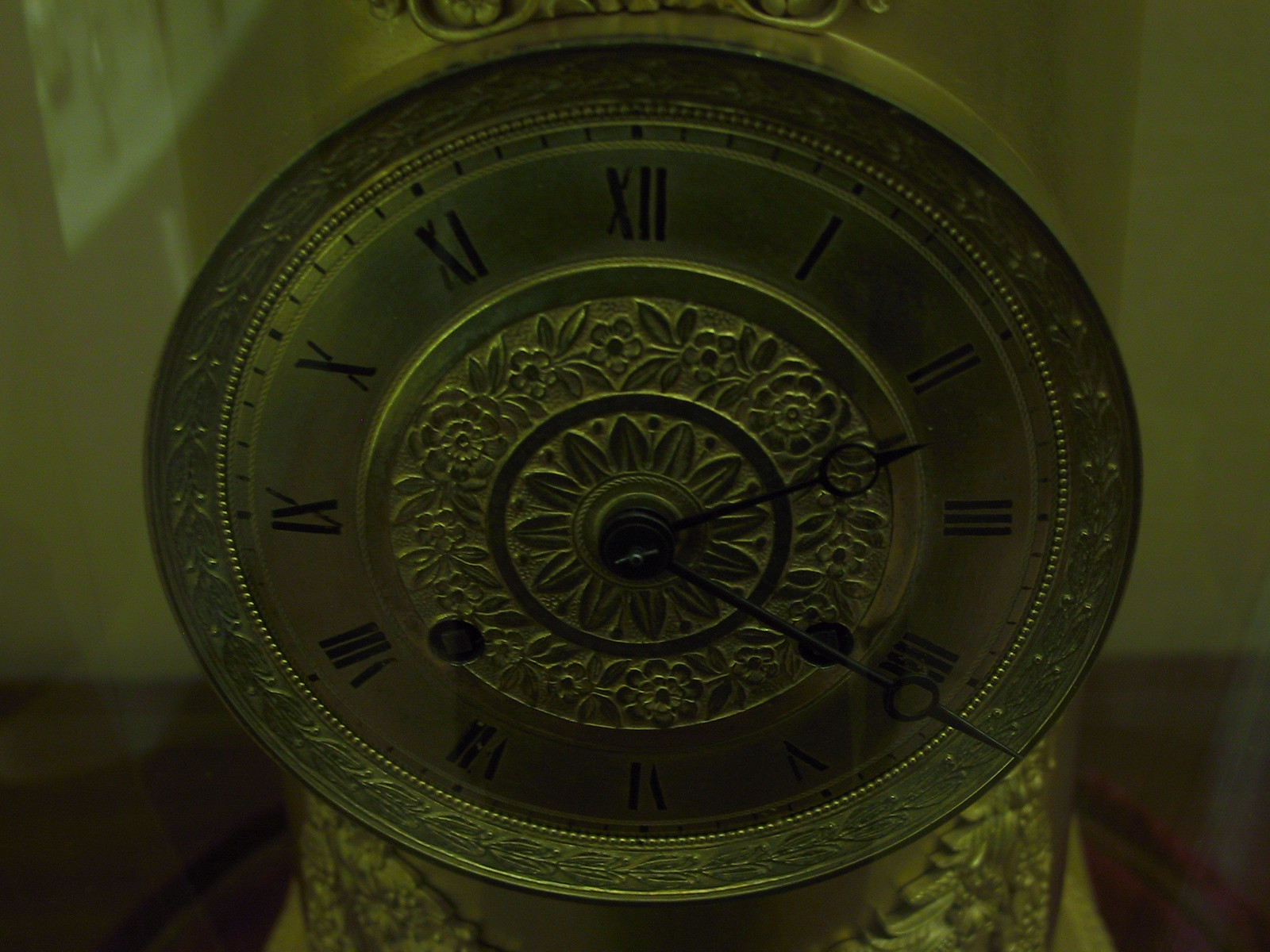This close-up photograph captures an ornately designed clock face, sharply detailed at its lower edge where it stands on a partially visible, intricate base. The centerpiece of the clock face is a floral motif around which the clock hands are attached. The face is adorned with elaborate floral patterns, and the hours are marked by black Roman numerals. An elegant design frames the outer edge of the clock face, further enriching its classical appearance. At the top, there seems to be an additional element, possibly made of bronze, although much of it is cut off in the photograph. The entire image possesses a greenish tint, adding a unique tone to the perceived bronze and black elements of the timepiece.